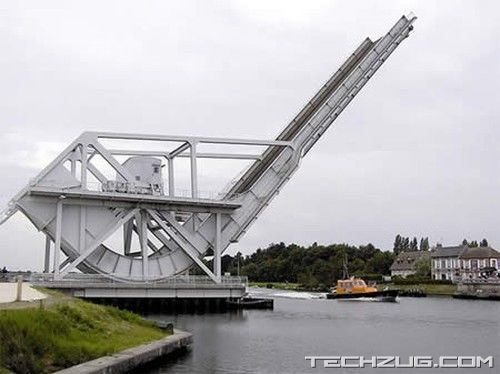The photograph captures a dramatic scene of a gray metal drawbridge raised to allow passage beneath it. The bridge, prominently positioned left of center, reveals only its elevated half, showcasing its intricate mechanical structure against a cloudy, rain-threatening gray sky. Below, the river mirrors the somber tones of the sky, its gray waters parting for a sizable black boat with an orange cabin navigating onward. To the right of the image lies a tranquil setting: a large two-story house sits behind a patch of trees, suggesting either a mansion or a guesthouse. The right-center of the image frames the opposite side of the river with a slight grassy area encircled by concrete. Overlaid on the bottom right corner of the image is the white text "TECHZUG.COM." The overall setting is a blend of industrial might and serene habitation, marked by differing shades of gray, green, orange, and black that accentuate its depth and complexity.